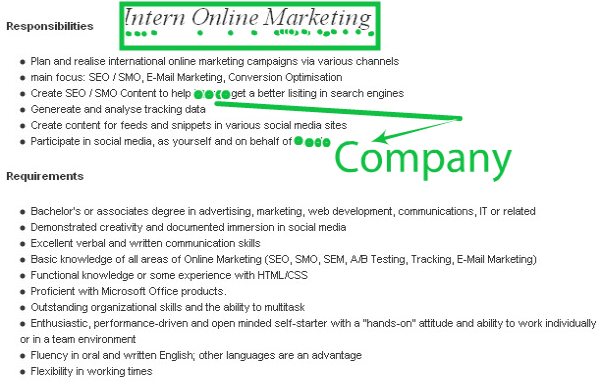This image features a screenshot of a job listing with a clean white background and predominantly black text, accented by some green highlights. The title at the top, "Intern - Online Marketing," is prominently displayed within a green rectangular border. Below the title, there are a series of green dots, seemingly placed by random clicks of the cursor.

The job listing is divided into two main sections: Responsibilities and Requirements. 

**Responsibilities:**
- There are six bullet points listed under this section. 
- The third bullet point reads: "Create SEO/SMO content to help [Company] get a better listing in the company engines." The name of the company is obscured by four green dots. A green zigzag arrow extends from this point to another area marked by four green dots and the word "company," all highlighted in green.
- The final bullet point states: "Participate in social media as yourself and on behalf of [Company]." Similar to before, the company's name here is covered with green dots.

**Requirements:**
- This section consists of ten bullet points, but the specific text of these points is not detailed here.

The green highlights and the dots used to obscure certain elements indicate sensitive information, such as the company's name, has been intentionally hidden in this screenshot.